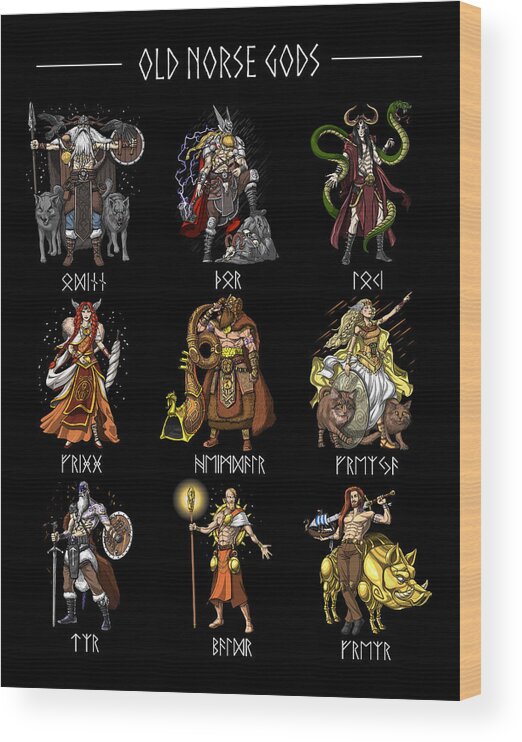This is a screenshot of a video game featuring a character selection page showcasing prominent old Norse gods. Displayed on a white background resembling a canvas with wood-textured sides, the central area is black with "Old Norse gods" written in thin white text at the top. 

Nine detailed figures are depicted, each with descriptive text and symbols beneath them. The first is an old man with a long white beard, holding a spear and shield, flanked by two gray wolves. Next is Thor, recognizable by his muscular build, silver winged helmet, red cape, and iconic hammer, standing with his foot on a rock. The third character, possibly Medusa, is a woman with two snakes emerging from her head, dressed in red. Further characters include a wizard with a snake behind his back, a princess with animal ears, a figure with a large trumpet, a princess accompanied by two cats, a warrior armed with a shield and sword, a wizard wielding a glowing staff, and another fighter brandishing a sword with a golden boar by his side.